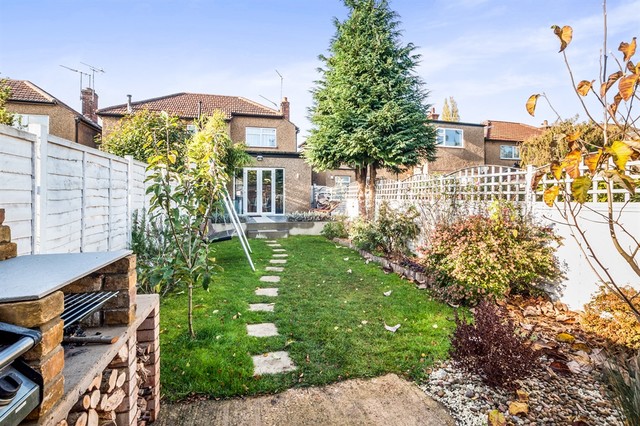The image depicts a quaint, narrow backyard garden in what appears to be a European neighborhood. Dominating the left side of the photo is a firewood grill, which could be used for barbecuing or making pizzas. A pile of logs is neatly stowed underneath the grill, indicating it's ready for use. Adjacent to the firewood grill, a wooden workbench can be spotted, further enhancing the outdoor cooking area.

The center of the yard features a brick walkway composed of square stone steps that create a path leading directly to the entrance of a brick, two-floor bungalow-type house. The entrance boasts triple glass panes, likely part of a patio door. On either side of the walkway, the garden is framed by white fences. The right fence is a mix of solid panels and open trestles, while the left fence is completely solid. Both fences are adorned with shrubbery, with the right side featuring mostly gray-green shrubs and a small tree close to the house. Left-side greenery includes small trees and shrubs, adding to the garden's lush feel.

Not far from the walkway's entrance on the left side is another barbecue grill, barely visible but adding to the yard's outdoor cooking amenities. The entire garden area is covered with a well-maintained, albeit slightly unclean, grassy lawn with a few tiled paths indicating where to walk. The view of adjacent brick homes suggests a cozy, community-centered neighborhood.